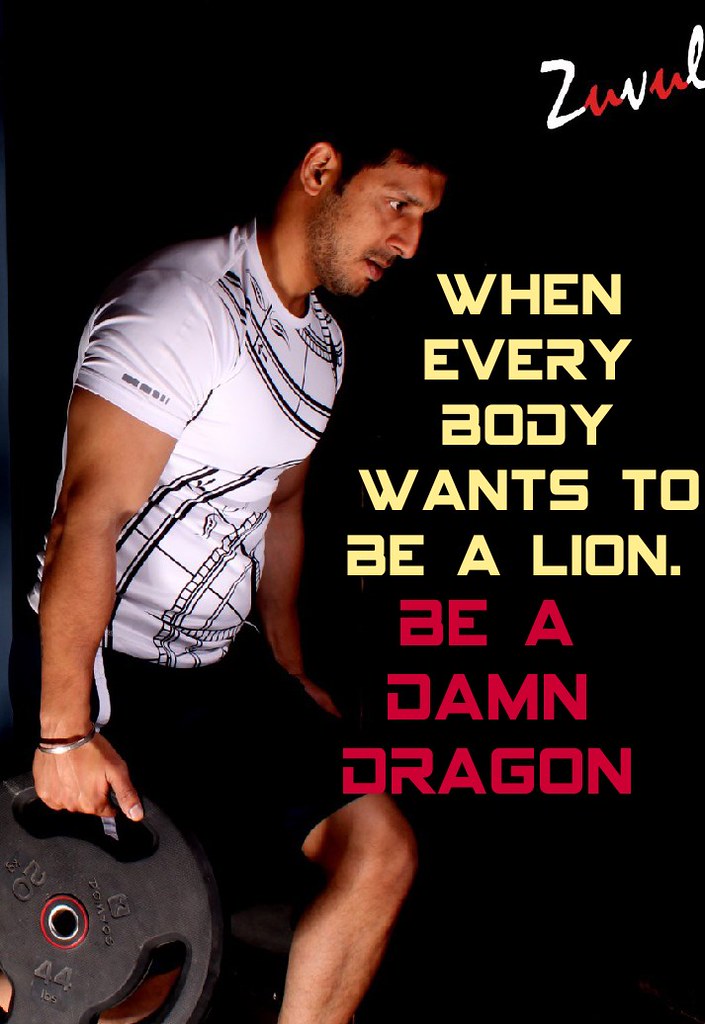The image depicts a man working out on the left side, wearing a white t-shirt adorned with various lines, and black shorts. He has brown hair, a hint of facial hair, and is holding circular weight plates with both his hands, each featuring a central opening and numbers inscribed. The weight plates are black and labeled “Zuvul,” with the letters transitioning from white to red. Prominently displayed on the right side of the image, in bold text, is the motivational phrase: "When everybody wants to be a lion, be a damn dragon." The words "everybody wants to be a lion" are in yellow uppercase font, while "be a damn dragon" is in red. All this is set against a stark black background, which emphasizes the man and the text.